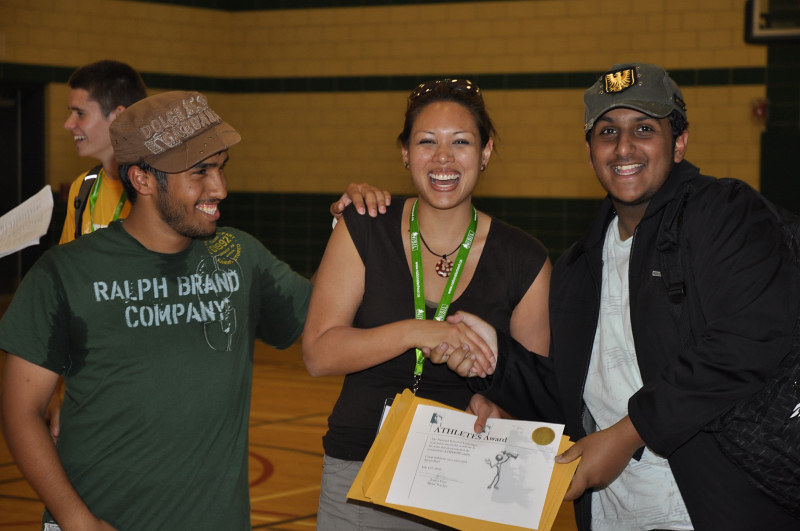In the indoor setting of a gymnasium with hardwood flooring painted for sports, likely a basketball court, three close friends are celebrating an achievement. The backdrop features a stone brick wall, lending a sense of solidity to the space. The central figure, a woman with light brown skin, stands proudly holding a certificate titled "Athletes Award," while beaming with a large smile. She wears sunglasses perched atop her head, a green lanyard, and a black sleeveless shirt. To her left, a man with darker complexion, dressed in a Ralph Brand company green shirt and a brown hat, places a supportive hand on her shoulder. On her right, another man with a gray baseball cap adorned with a gold bird and a black hoodie over a white undershirt, steadies the certificate with his left hand while shaking her hand. Both men are smiling warmly, perhaps reflecting shared joy and pride in her accomplishment. Behind them, slightly out of focus, stands another gentleman also smiling, adding to the atmosphere of celebration and camaraderie. The image is vibrant, with colors spanning black, tan, green, yellow, light green, gray, and gold, capturing a moment of triumph and togetherness.